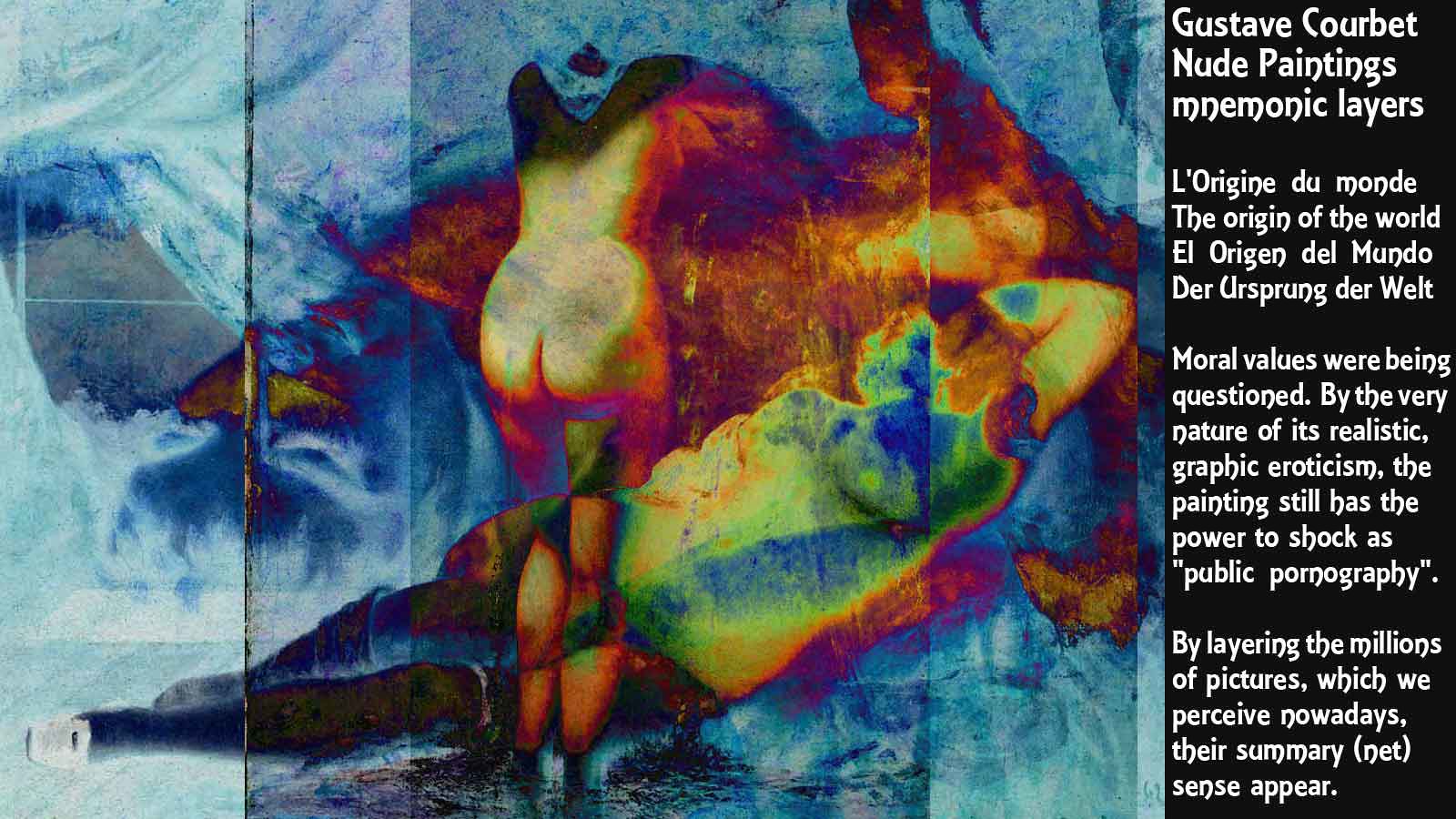The image features an abstract painting of a nude woman seen from behind, depicted without a head as she appears to be bending over. The painting is richly textured with an array of colors including blues, greens, yellows, reds, and purples, with the corners predominantly shaded in varying tones of blue. To the right of the painting, a vertical black rectangle contains white text that reads "Gustave Courbet, Nude Paintings, Mnemonic Layers." Below this title, the text "L'Origine du Monde" (The Origin of the World) is present, suggesting the painting’s name. Additional text in both English and French comments on the controversial nature of the artwork: "Moral values were being questioned by the very nature of its realistic graphic eroticism. The painting still has the power to shock as public pornography. By layering the millions of pictures which we perceive nowadays, their summary sense appear." This commentary highlights the painting's ability to provoke and its lasting impact on viewers through the evocative use of modern visual elements and colors.